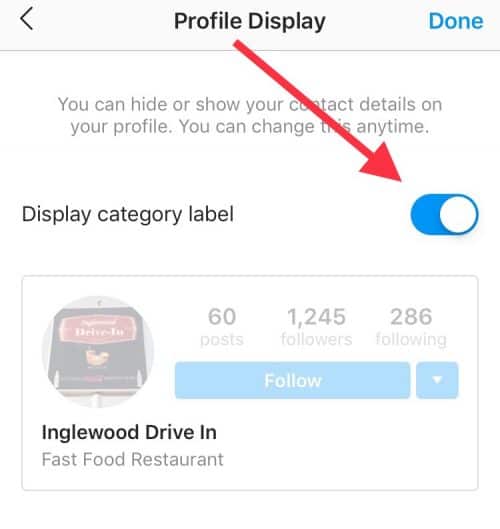In the middle of the upper edge of the screen, there is a black profile display. To the left and right of this profile, there are arrows pointing in their respective directions. A blue "Done" button is also located to the right. From the profile display, a red arrow points towards a toggle switch. Left of this toggle switch, there is a label that reads "Display Category Label." Below the profile display, a note says, "You can hide or show your contact details on your profile. You can change this at any time." The user has opted to turn on the "Display Category Label."

Below this section, there is a horizontally extended rectangular card with the following information:
- "Englewood Drive-in fast-food restaurant"
- "60 posts"
- "1245 followers"
- "186 following"

The card also features a "Follow" button and a downward drop-down arrow, which is grayed out. The entire card has a light hazy appearance with a gray border around it. The color scheme in the image includes black, white, teal blue, gray, red, blue, and yellow. The Englewood Drive-in's logo is present but not clearly visible due to being grayed over.